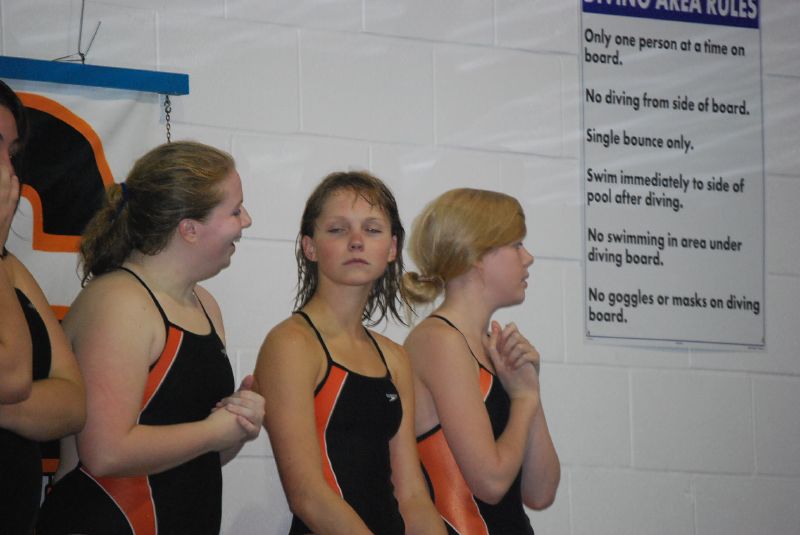In this detailed photo description, we find three young ladies, likely high school swimmers, standing in front of a white, cinder block wall adorned with swimming area rules and their team's black and orange logo. All three girls donn identical black swimsuits featuring striking orange stripes down the sides. The girl on the right has blonde hair and is posing with her hands held up under her chin. The girl in the middle, with longer brownish-reddish hair, gazes toward the camera with her eyes nearly closed. She is engaged in a light-hearted conversation with the third girl, who appears to be laughing. This third girl, slightly larger in stature, is also in the same colorful team swimsuit. Above them, prominently displayed, are pool safety rules such as "one person at a time on the diving board," "no diving from the side," "pool bounce only," "swim immediately to the side after diving," "no swimming under the board," and "no goggles or masks on the diving board." The girls seem to be in a candid moment, possibly waiting their turn to dive in the indoor swimming pool.